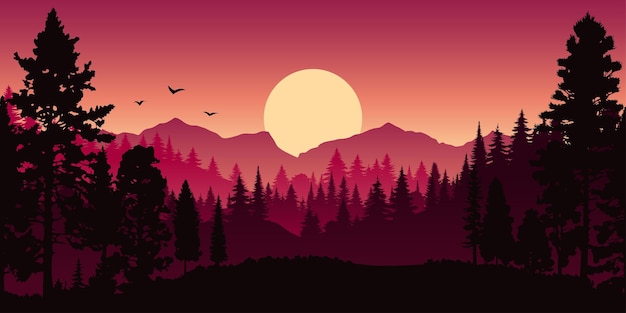This 2D cartoon-style illustration depicts a mesmerizing sunset scene with a gradient sky transitioning from magenta and pale peach at the top to deep purple and black at the bottom. Dominating the center of the image is a large, off-white, yellowish sun that bathes the landscape in warm hues. Below the sun lies a layered mountain range, which starts with pinkish-red tones closest to the sun and fades to darker reds as it extends outward. Nestled at the base of these mountains are fir trees that transform in color; those farthest from the viewer are almost black, creating a stark silhouette against the fading light, while those nearer adopt purplish and hot pink shades. Three black birds, rendered as small 'V' shapes, appear to be soaring towards the sun, adding a dynamic touch to the tranquil scene. The dark shadowed trees are mainly positioned on the sides, framing the vivid, almost surreal landscape that captures the essence of twilight descending upon a serene wilderness.